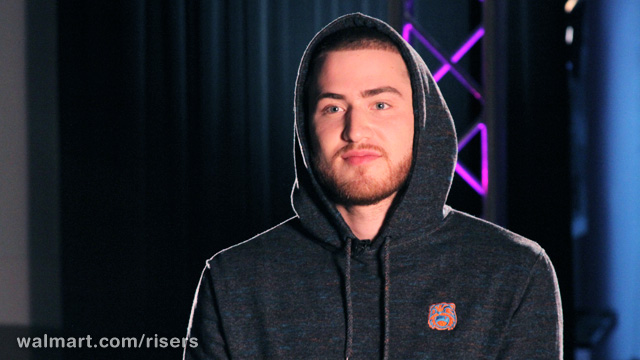The image portrays singer and songwriter-producer Mike Posner against a dark, stage-like background. Posner, occupying the right side of the frame, is dressed in a hooded gray tweed sweatshirt. The hood is pulled up over his closely trimmed, short dark brown hair, which features a faint white line across his forehead. His thick dark eyebrows slightly raised, he gazes neutrally off to the left. His light-colored eyes and dark brown beard with a mustache add to his distinct appearance. The sweatshirt features an emblem on the chest, depicting an animated cow with a mix of orange, blue, and dark blue colors. Dangling bands or ties from the hoodie hang down the front. The backdrop includes a mix of dark gray drapes, a vertical light gray band, and purple decorative towers or risers with some blue accents, giving the impression of a stage setting. In the bottom left corner, the text "walmart.com/risers" is subtly displayed in light gray against the dark background.